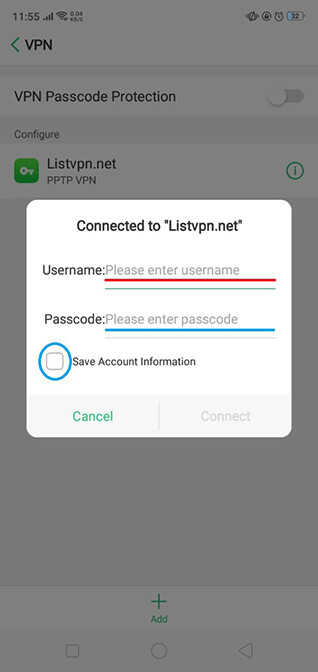The image depicts a cell phone screen displaying a VPN configuration interface. The battery level is at 22%, and the signal strength shows 5 bars. The main screen has a gray overlay, indicating a focus on VPN passcode protection. An overlay reads: "VPN Passcode Protection. Configure ListVPN.net PPT VPN."

In the foreground, a white pop-up window is prompting the user to connect to ListVPN.net. The window has fields for entering a username and passcode, both currently blank. The "Username" field is preceded by a red bar, while the "Passcode" field is highlighted with a blue bar. Beneath these fields is a checkbox, encircled in blue, with the option to "Save account information."

At the bottom of the pop-up, there are two buttons: "Cancel," which is gray with green font, and "Connect," which is also gray but with gray font. The screen utilizes a color palette of green, gray, black, red, blue, and white. It is evident that the user is attempting to input new VPN information to connect to the ListVPN.net network, as there are no pre-saved VPN configurations displayed.